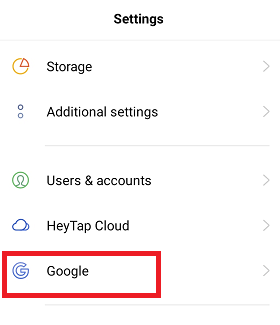A detailed screenshot of a settings page on a mobile phone application. The background is white. At the top center, bold black text reads "Settings," with the 'S' capitalized and the rest in lowercase letters. A thin light gray line is positioned directly underneath this title. Below this line, there are two sections of smaller black text accompanied by icons on the left and arrows on the right, which are light gray and point to the right.

The left-aligned icons are distinct and visually descriptive:
1. The first icon has a thin yellow outline with a red outlined slice cut out of it. To the right of this icon, the text reads "Storage."
2. The second icon consists of two blue outlined dots. To its right, the text reads "Additional Settings."

Following these sections is another thin light gray line, which does not extend fully to the left edge of the page. Below this line are three additional settings, each with unique icons, listed from top to bottom:
1. A green profile picture icon corresponds to the "Users and Accounts" setting.
2. A blue cloud icon corresponds to the "Haytap Cloud" setting.
3. A blue outlined 'G' icon corresponds to the "Google" setting, both of which are surrounded by a red box for emphasis.

This meticulous layout illustrates the structured design and various options available within the settings page of the mobile application.